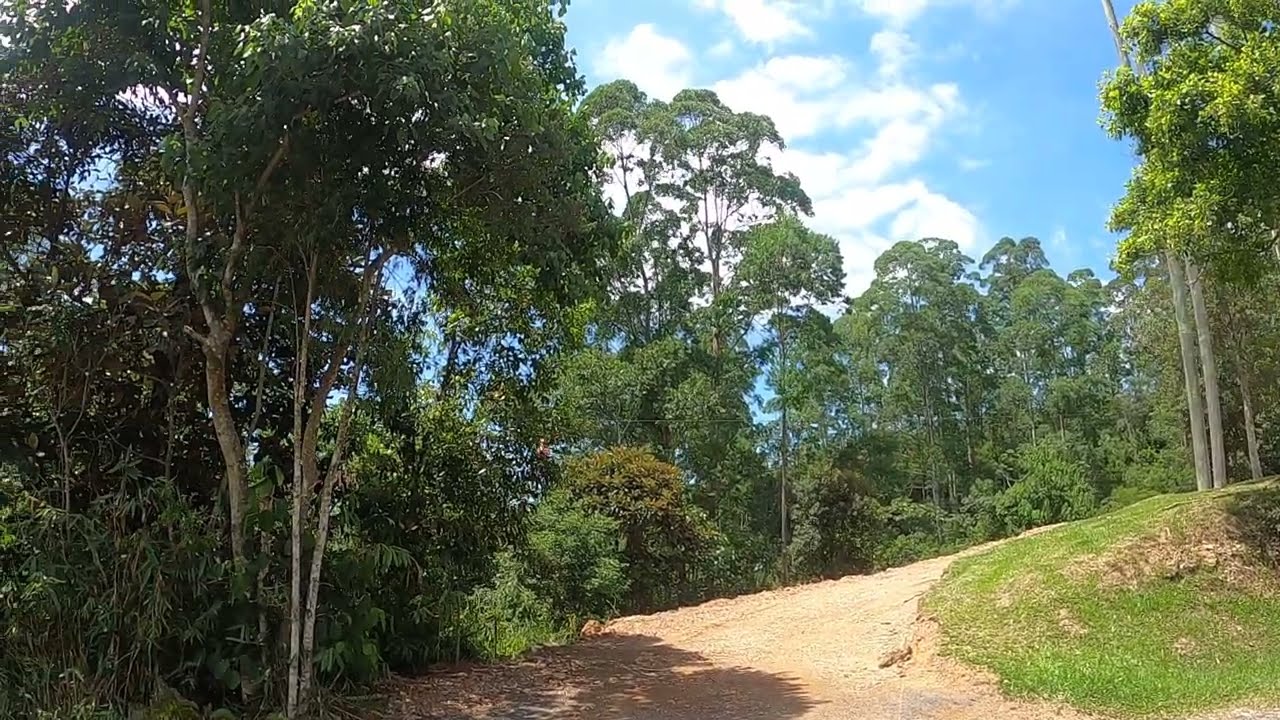The photograph captures a vibrant landscape featuring a winding dirt trail emerging from the lower middle and curving to the right, disappearing behind a small grassy hill. The grass, located predominately in the lower right quadrant, is a vivid green. Left of the trail, a dense assembly of trees with bright green foliage and brownish-gray trunks extends upwards, casting shadows on the pathway beneath. 

The scene is illuminated by sunlight coming from the left, creating dappled light effects on the verdant leaves and darker shading under the trees. In the background, a mixture of tall and medium-sized trees further complements the landscape, with their branches revealing glimpses of a mostly cloudy sky showing patches of light blue. The upper right corner of the image is especially noteworthy as it showcases the sun-lit leaves against the sky.

Overall, the image beautifully balances the interplay of light and shadow, accentuating the diverse shades of green and capturing the tranquil essence of this picturesque landscape.